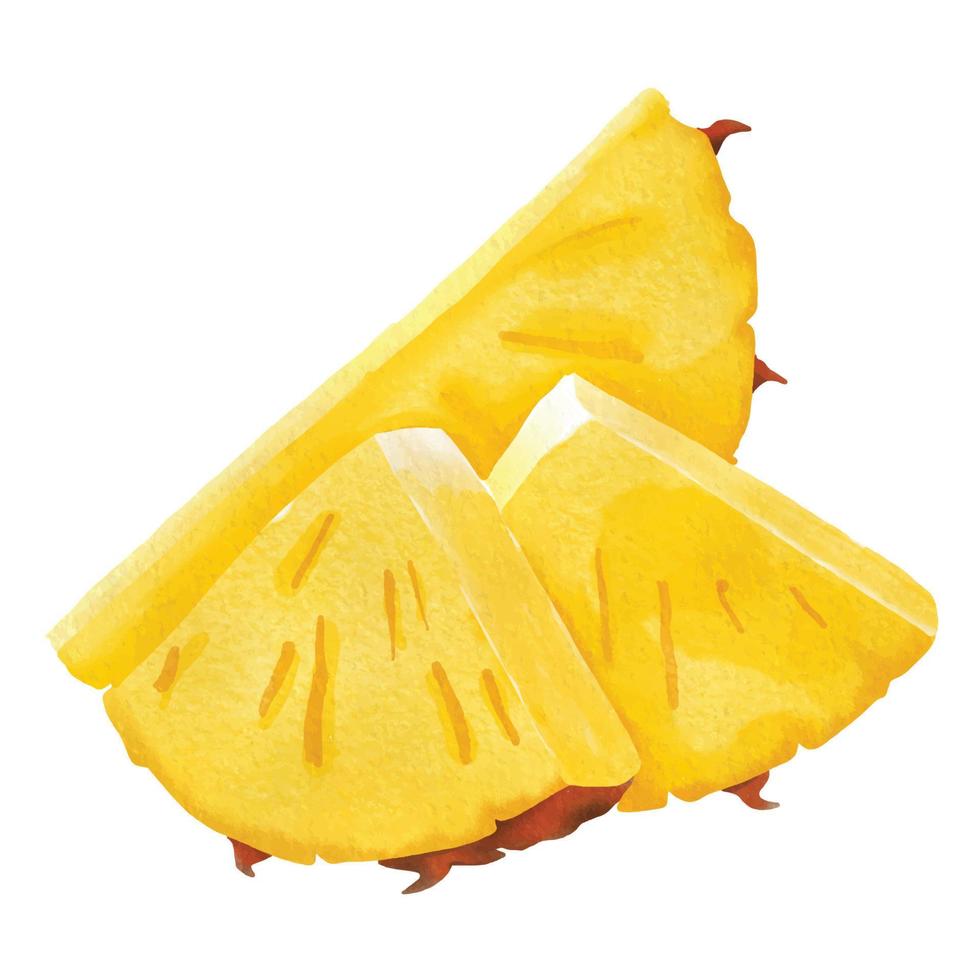This detailed watercolor illustration showcases three pieces of pineapple against a plain white background. In the foreground, two overlapping wedges display their yellowish-gold flesh, with the skin still attached on the curved bottom sides. The edges of the fruit slightly lighten, suggesting highlights from a light source. One of the foreground wedges is elongated, while the other leans at an angle, both featuring the characteristic brown pointy spots of the skin. Behind these wedges, a larger slice shaped like a quarter circle, also yellowish-gold with brown spikes, sits prominently. The watercolor technique gives the image a soft, slightly abstract quality while capturing the texture and detail of the pineapple, highlighting its realistic appearance despite being a painting.